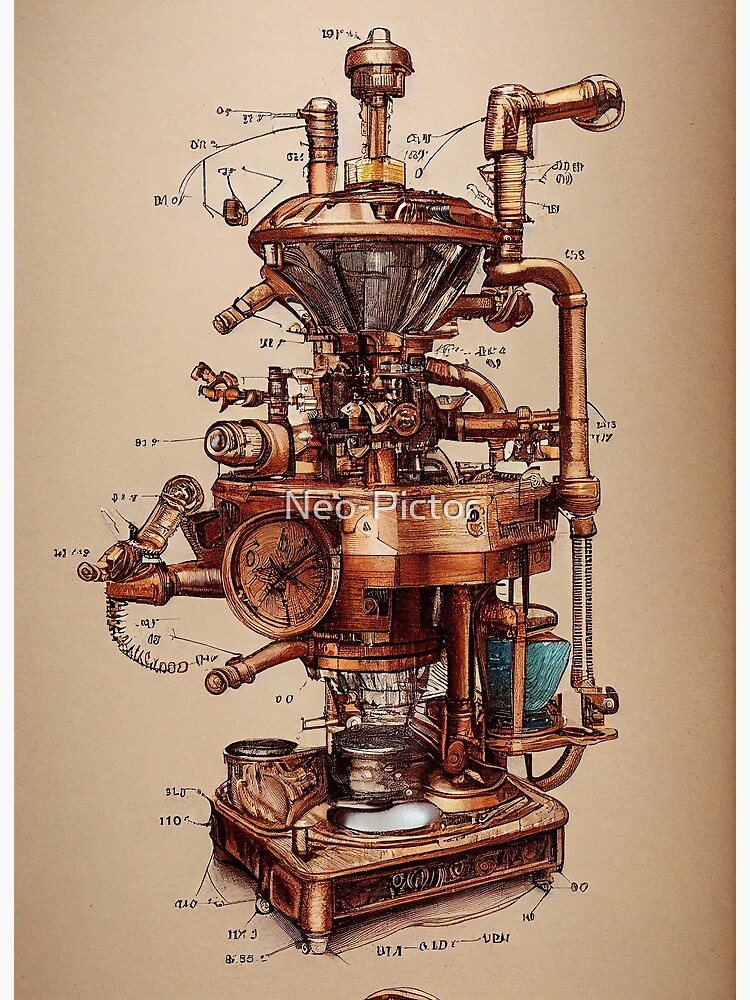This hand-drawn illustration, accentuated with pen and ink and colored pencils, depicts a tall, steampunk-inspired, mechanical device set against a tan-brown background. The contraption, which exudes a brass-steel appearance with copper tubes and valves, seems reminiscent of an antique cappuccino machine or a complex piece of machinery. It features a square base that transitions into a cylindrical shape, widens into another square form at the middle, and then tapers again towards the top. The structure is adorned with numerous gauges, screws, pipes, and dials, likely for measuring pressure (PSI) and other metrics. Surrounding the device, there are multiple black dashes, numbers, text, and symbols with arrows pointing to different parts, potentially explaining each component. Centrally overlaid on the image is a white watermark with the partly distorted text “NEO-PICTOR” or “Neo-PictoC.”